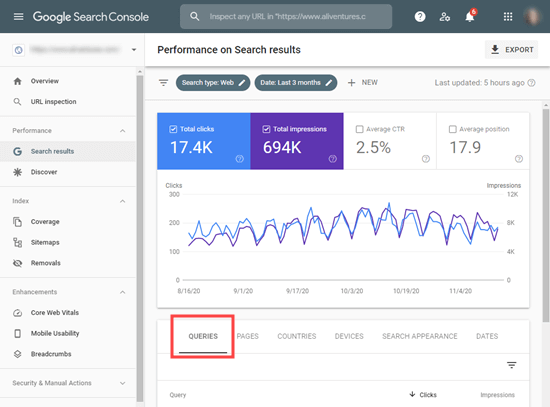This screenshot showcases a Google Search Console page with a predominantly off-white background. At the top, a charcoal gray header bar features several elements positioned from left to right. Initially, the header displays "Google Search Console" in white text. To the right, there is an extended gray search bar with white text that includes a magnifying glass icon on the left, followed by the text "Inspect any URL," and an example URL "https://www.allventures.c." This is succeeded by a white circle containing a question mark, a user icon depicting a head and shoulders silhouette, and a notification bell icon.

Centered below the header, the title "Performance on Search Results" is prominent. Adjacent to it, on the right side, there is a downward-pointing directional arrow and an "Export" button. 

The left side of the interface features a vertical rectangular menu listing multiple options: "Overview," "URL Inspection," "Performance," "Search Results," "Discover," "Index," "Coverage," "Sitemaps," "Removals," "Enhancements," "Core Web Vitals," "Mobile Usability," "Breadcrumbs," "Security," and "Manual Actions."

In the main section towards the center-right, two ovular bubbles display key statuses. The first bubble states "Search Type: Web," and the second bubble presents "Date: Last 3 months," followed by a "+ New" button and a timestamp indicating "Last updated: 5 hours ago."

Below this section, four square boxes relay performance metrics. The first box, colored blue with white text, reads "Total Clicks: 17.4k." Next, a purple square displays "Total Impressions: 694k." Following these, a white box shows "Average CTR: 2.5%," and another white box presents "Average Position: 17.9."

A graphical representation of the data lies beneath these performance metrics, followed by tabs categorizing further details under "Queries," "Pages," "Countries," "Devices," "Search Appearance," and "Dates."